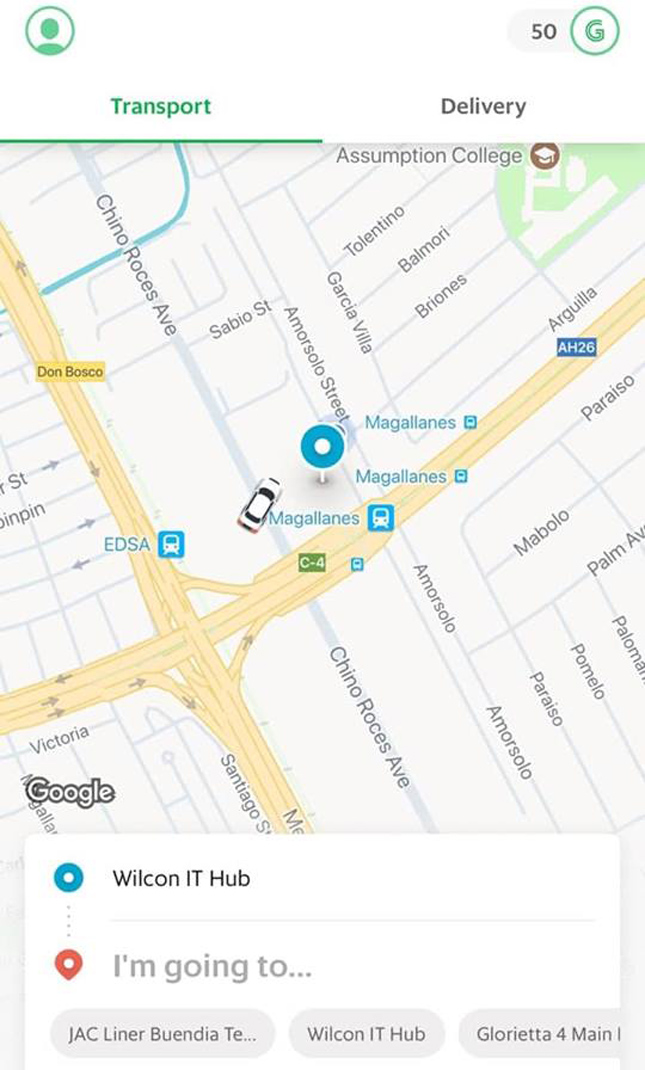The image features a white background with various colorful elements and text. Central to the composition is a blue circle containing a green icon representing a person’s head and shoulders. Adjacent to this is a depiction of transportation in green and delivery in black. Nearby, a small rounded box contains the number "50."

A green circle with a green "G" inside it and a horizontal green line about halfway across the image are also present. A map prominently displays the name "Assumption College" at the top, with "Don Bosco" highlighted in a yellow box. 

Further details include a labeled road, "EDSA," a blue box featuring a bus, and multiple mentions of "Mega Lanes," alongside a car illustration. One of the "Mega Lanes" is highlighted by a white circle with blue and white layers inside. 

At the bottom, the word "Google" appears in white letters outlined in black. An inset box, white with a blue circle containing white inside it, reads "Wilcon IT Hub." Blue dots lead to a red circle with white interior text reading "I'm going to," followed by ellipses and three gray boxes listing "JAC Liner Buendia," "Wilcon IT Hub," and "Glorietta for Maine."